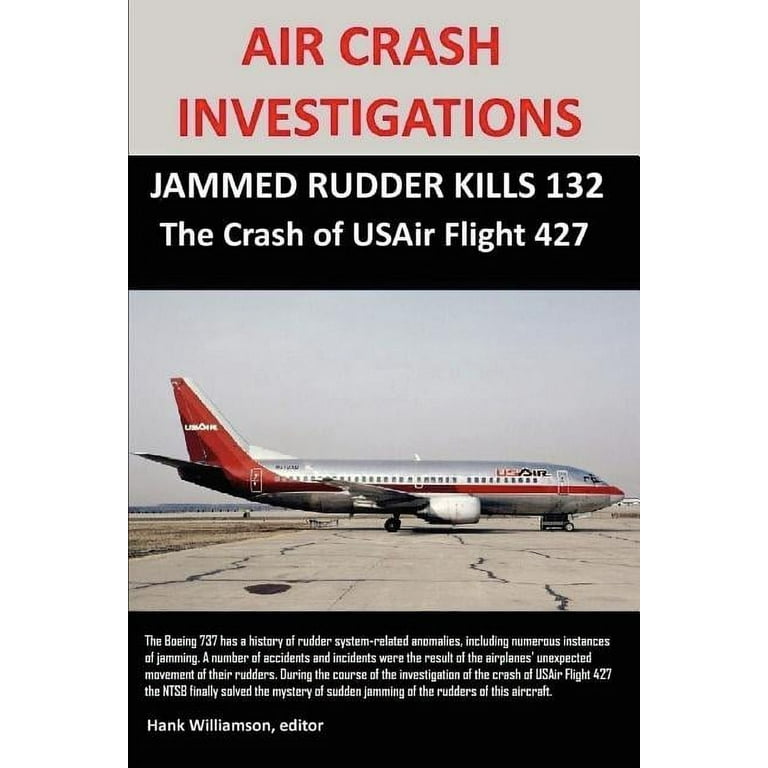The document appears to be the cover page of an investigative report titled "Air Crash Investigations." The main title is prominently displayed in red letters on a gray background, and below it, in white text on a black band, is the subtitle "Jammed Rudder Kills 132: The Crash of U.S. Air Flight 427." Central to the page is a photograph of a large, silver airplane adorned with red stripes and a red tail, clearly marked "U.S. Air." The plane is positioned on a cracked tarmac, showcasing a side view that emphasizes its size, complete with rows of windows and a single visible door.

Below the photograph, the document details historical issues with the Boeing 737's rudder system, mentioning numerous instances of jamming, unexpected movements, and resultant accidents. The report explains how the NTSB's investigation into U.S. Air Flight 427 eventually unraveled the mystery behind the rudder malfunctions. At the very bottom, the document credits Hank Williamson as the editor of the report, connecting him to the thorough explanation of the rudder system anomalies.